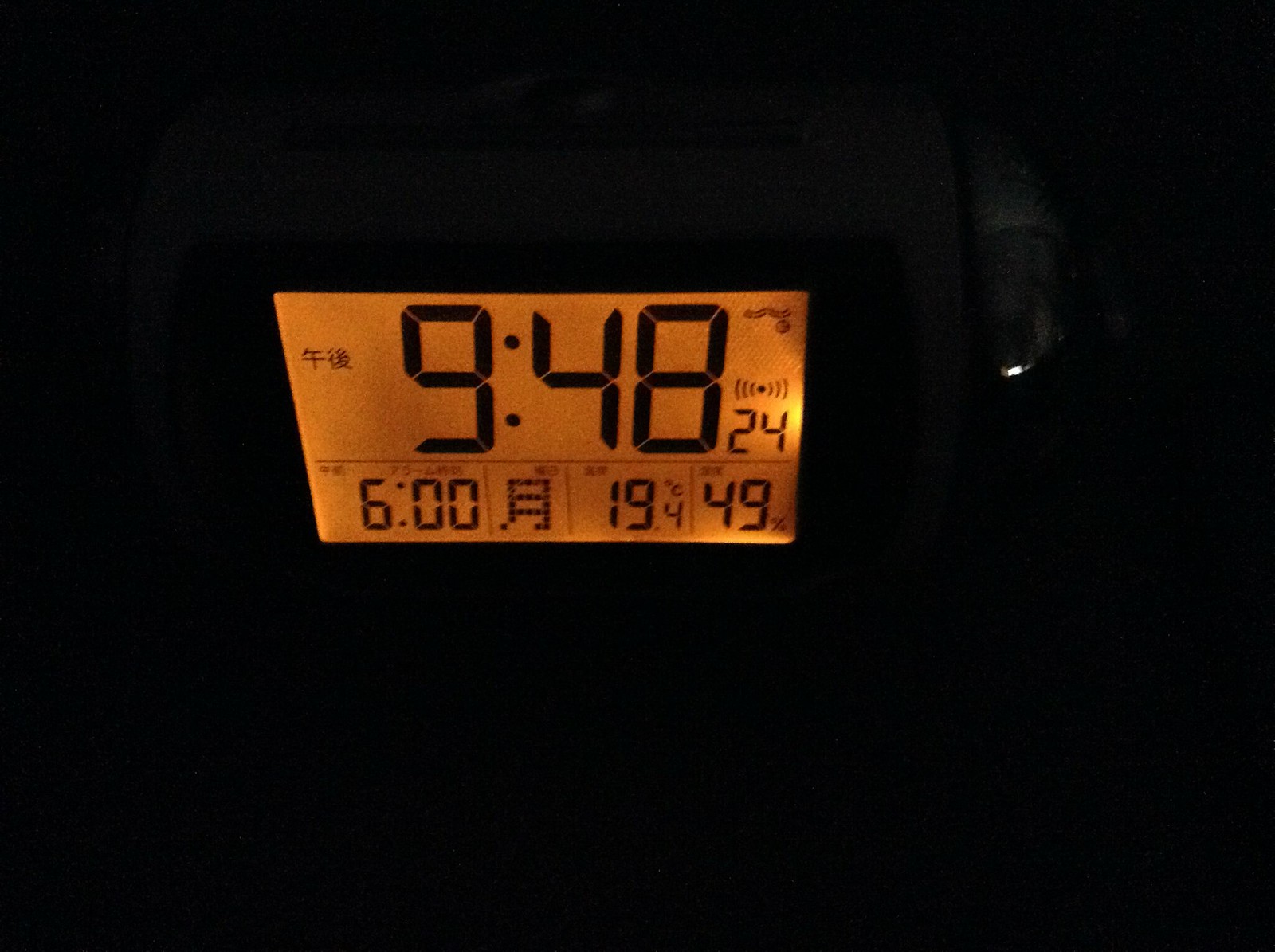This image features a rectangular electronic clock face prominently set against a dark, nearly black, background. The clock, encased within a dark ring, emits a soft orange glow. The display shows the time "9:48" along with the figure "24," likely indicating seconds or military time. Above the "24" is a Wi-Fi symbol. Notably, the clock includes Chinese characters, suggesting it might be a clock from China. The clock lists "6 o'clock" and has another Chinese character in the lower left corner. The digital display also indicates "19.4" and "49%," which could relate to percentages or some other measurement. On the right-hand side, a secondary whiteish-grey glow is visible, though it is unclear whether this is part of the clock or an external element.